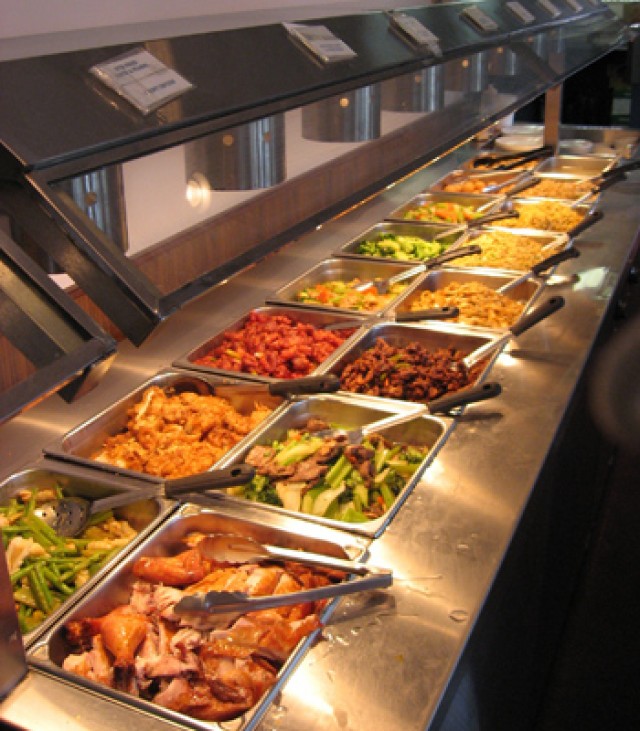The photograph captures a slightly blurry view of a buffet line from the server's perspective, showcasing a total of 16 metal trays organized in an 8 by 2 layout under warming lamps. Each tray is filled with various types of food, including chicken, green beans, beef, broccoli, cauliflower, pasta, and possibly red peppers, with trays closer to the front more easily identifiable. The trays are equipped with appropriate serving utensils like metal spoons with black handles, slotted spoons, and tongs. At the very end of the line, there are stacks of white plates; two stacks consist of large plates while one stack has smaller plates. The buffet is enclosed by a sneeze guard, and atop it are small white labels, albeit not clearly legible due to the blurriness of the image. The setup evokes an industrial kitchen or a self-serve deli counter, similar to the style found in restaurants like Chipotle.